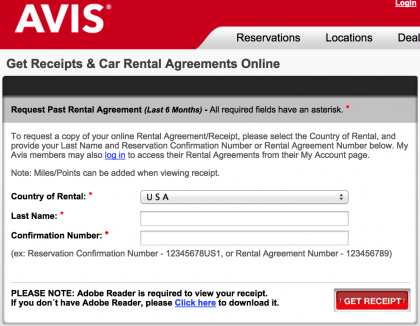Screenshot of a webpage with a white background featuring the Avis logo. The page includes options such as "Log In," "Reservations," "Locations," and "Deals." There is a section titled "Get Receipts and Car Rental Agreements Online," with the subtitle "Request Past Rental Agreement (Last Six Months)." All required fields are marked with a red asterisk.

The text instructs users to request a copy of their online rental agreement or receipt by selecting the country of rental and providing their last name along with their reservation confirmation number or rental agreement number. Avis My Account members can log in, with the "Log In" option highlighted in blue, to access rental agreements from their account page. There is a note indicating that Miles/Points can be added when viewing the receipt.

Fields displayed include "Country of Rental" marked with an asterisk and a drop-down showing "USA," "Last Name" marked with an asterisk with an empty input box, and "Confirmation Number" marked with an asterisk with an empty input box. An example format for the confirmation number is shown, indicating a series of numbers followed by three letters.

There is also a mention of an option to enter a rental agreement number, illustrated with a sample number.